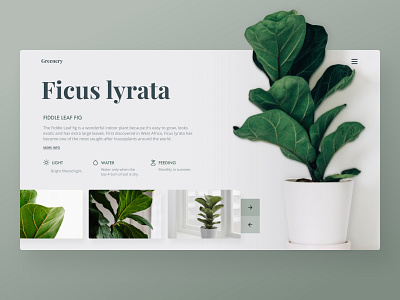The image features a digital design template set against a gray background, showcasing a white flower pot on the right containing a green plant with large, dark green leaves, identified as a Ficus lyrata, also known as a fiddle leaf fig. The plant's name "ficus lyrata" is written in black text on the left. The design mimics a website layout, complete with a menu button composed of three lines in the top right corner. Below the menu button is the plant illustration. At the bottom of the image are three smaller pictures: the leftmost displays a detailed view of the leaves, the middle highlights more of the plant, and the rightmost shows the entire plant situated in a more elaborate setting. Although the specifics are blurry and hard to read, the text seems to provide care instructions, likely detailing its light and water needs.